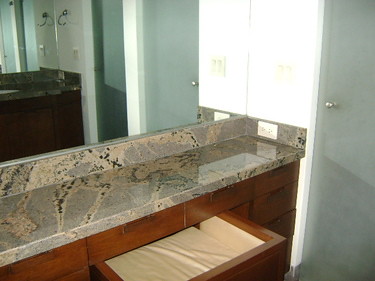In the photograph, we see a narrow bathroom counter adorned with a luxurious greenish marble countertop. Below the countertop, there is cabinetry made of dark wood featuring multiple drawers, with one drawer partially open to reveal a piece of white fabric inside. 

Above the counter is a short backsplash matching the green marble, which adds a cohesive touch to the design. Rising from the backsplash is an expansive mirror covering the entire wall, creating an illusion of space and reflecting various elements in the room.

To the right of the scene, a white wall hosts a couple of switches, and just below this, there is an electrical outlet embedded in the backsplash. Further to the right, a light greenish door stands partially open, and its reflection is visible in the large mirror. Adjacent to this door, another doorway is discernible in the background, adding depth to the composition.